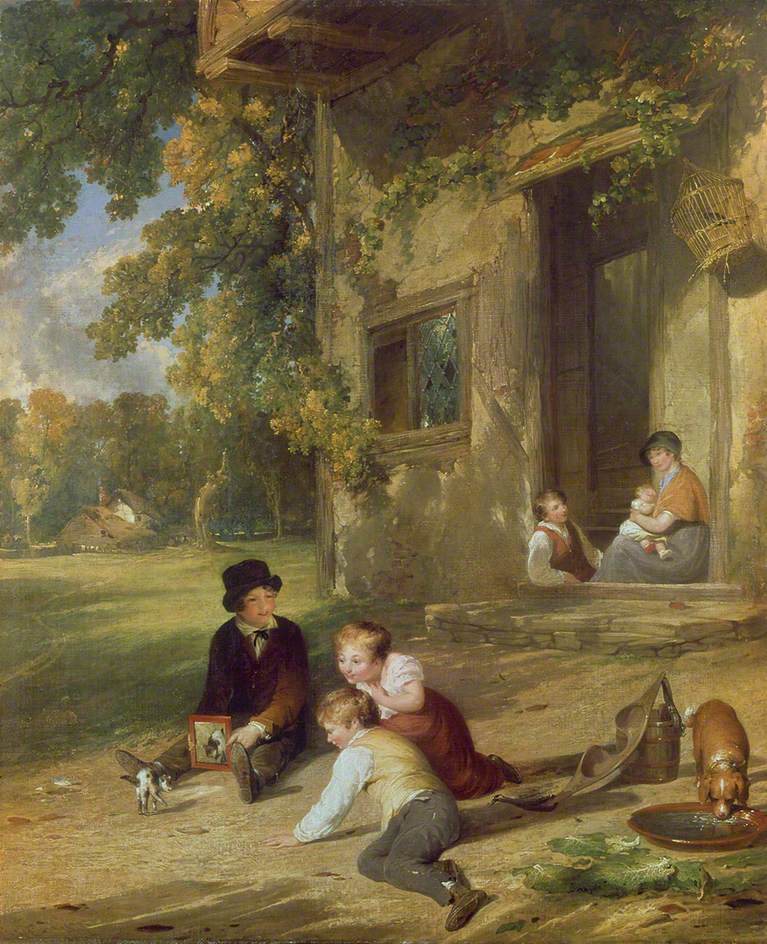This detailed oil painting, titled "The Kitten Deceived" by William Collins from 1816, is a vertical rectangular piece in the classical Victorian style with vivid, realistic lighting. The scene depicts a rustic front yard with a brown stucco house occupying the upper right portion. The house features a square window and a hanging basket near the door, which may house a bird. The door itself is made of dark brown wood.

At the doorway, a young woman sits on the porch steps with an infant in her arms. She is adorned in a dark bonnet, a gold or orange blouse, and a gray skirt. Leaning against the doorway is a young man wearing a long-sleeved white shirt and an orange or brown vest, gazing up at her.

The lower half of the painting captures three children playing. The boy on the left is outfitted in a top hat, a dark brown coat, and a bow tie, holding what may be a book or wooden object. The other two children, finely dressed in Victorian attire, are engaged with a small kitten. One child is holding a mirror up to the kitten, which approaches the reflection curiously. 

In the bottom right corner, a small dog, possibly a beagle, is drinking from a large brown water bowl, with a canister nearby. The background is adorned with lush green trees sporting golden leaves, adding a serene touch to the idyllic scene.